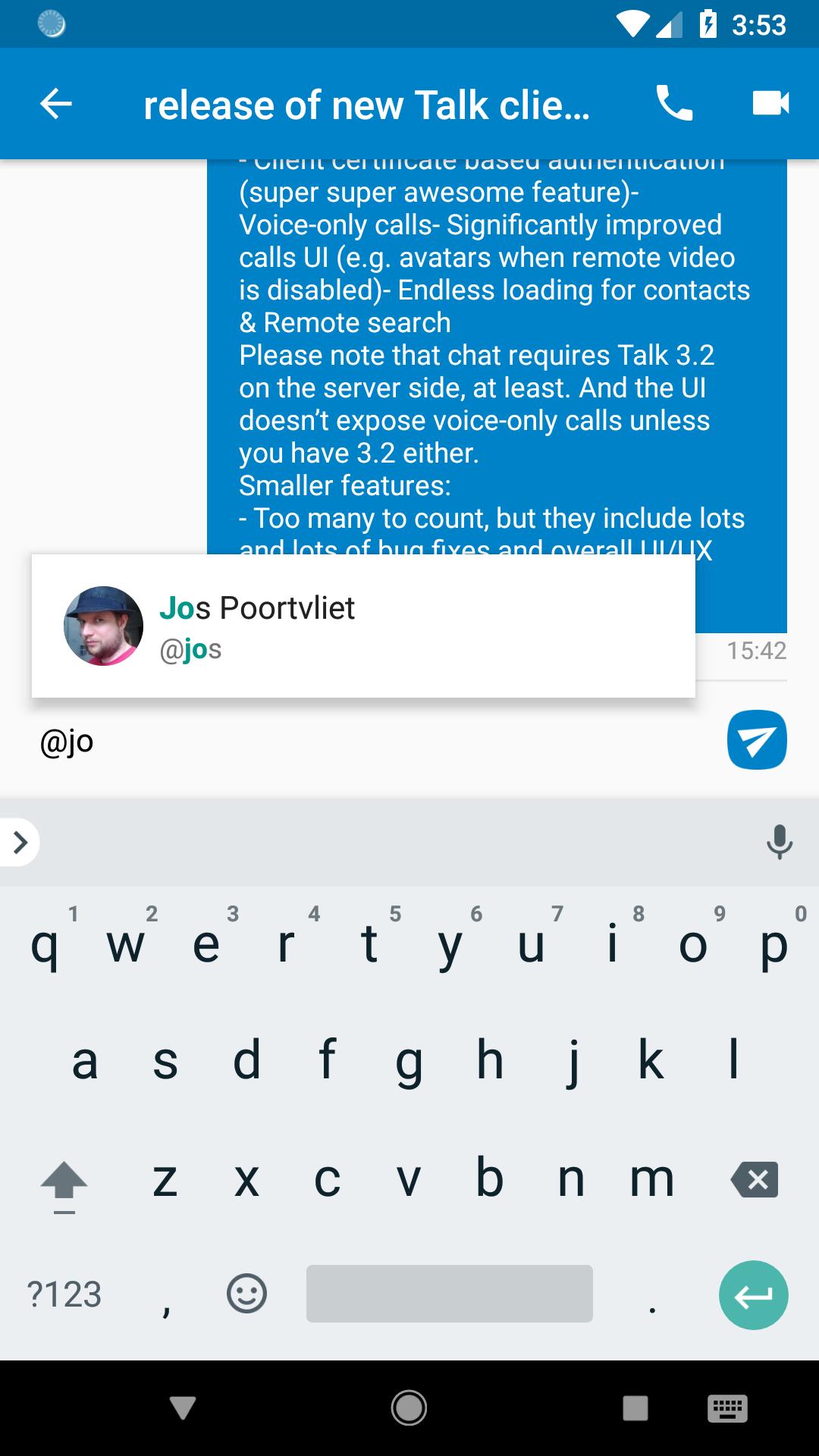A screenshot of a smartphone displaying a social media chat is captured in this image. The top right corner of the screen shows the current time at 3:53. Adjacent to the time, a vertical battery icon, featuring an electricity symbol, indicates that the phone is currently being charged. To the left of the battery icon, both the phone’s signal strength—displayed at about halfway—and a fully connected WiFi signal are visible. Centered at the top, the words “Release of New Talk, Ply…” are partially shown. On the left side of this text, there is a white arrow, while the right side features a phone icon and a camera icon, both in white on a blue background.

Midway down the image, there is a blue rectangle with a lengthy paragraph of white text. Beneath this, another white rectangle contains the name “J-O-S Port Relay,” accompanied on the left by a circular profile picture. The lower half of the image prominently displays the phone's keyboard interface. At the very bottom, a camera icon is positioned in the center, while a keyboard icon rests on the bottom right.